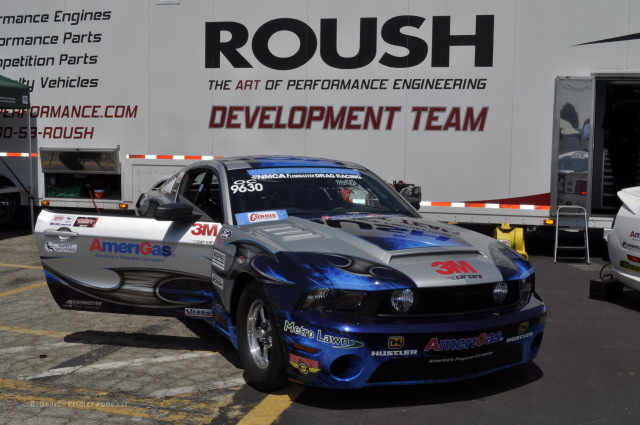This photograph depicts a blue and silver Ford Mustang race car, prominently positioned in front of an off-white building with the signage "Roush, The Art of Performance Engineering Development Team." The car, adorned with various sponsor logos including 3M, Amerigas, Hustler, and Metrolon, balances its metallic blue body with a slate gray hood and doors. The number "9630" is displayed on the windshield, and text referring to "drag racing" is faintly recognizable. While the car is clearly designed for high performance and developmental purposes, it is notably stationary with the passenger side door ajar, emphasizing its detailed setup against a backdrop that features additional text like "performance engines" and "competition parts." The scene is lit by daytime light, although the sky itself is not visible.